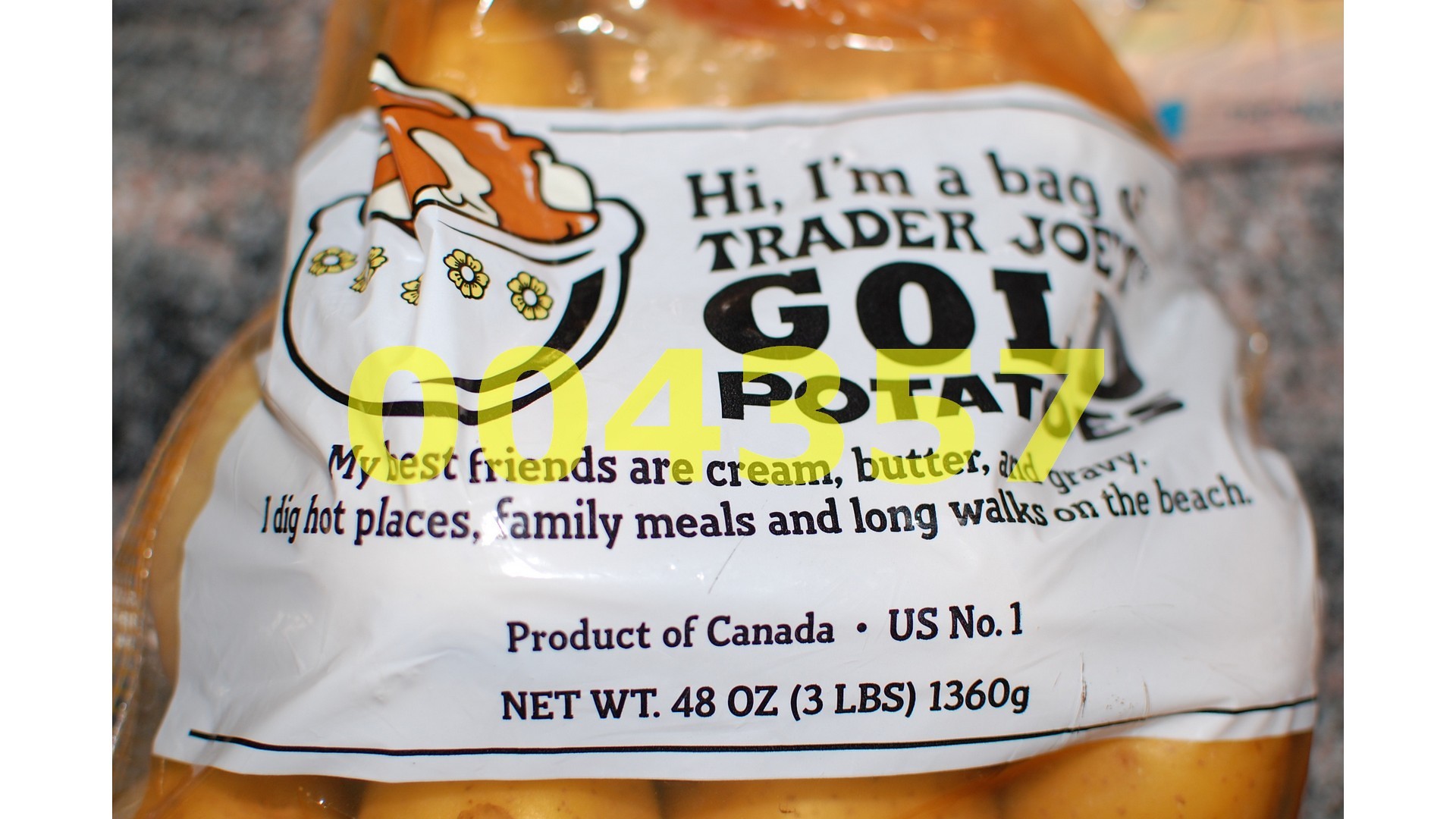The image depicts a plastic bag of Trader Joe's gold potatoes resting on a granite countertop, which has a mix of gray and pink tones. The bag is clear with an orangish tint, allowing a view of the medium golden-brown potatoes inside. A large white horizontal label is prominently featured on the bag. The label includes black text that reads, "Hi, I'm a bag of Trader Joe's GOLD potatoes. My best friends are cream, butter, and gravy. I dig hot places, family meals, and long walks on the beach." Beneath this, it states "Product of Canada, US number one, net weight 48 ounces, 1360 grams." In the upper left-hand corner of the label, there's an illustration of a white bowl with yellow flowers and brown contents, possibly cooked potatoes with steam rising. Superimposed in yellow numbers across the bag is the code "004357."